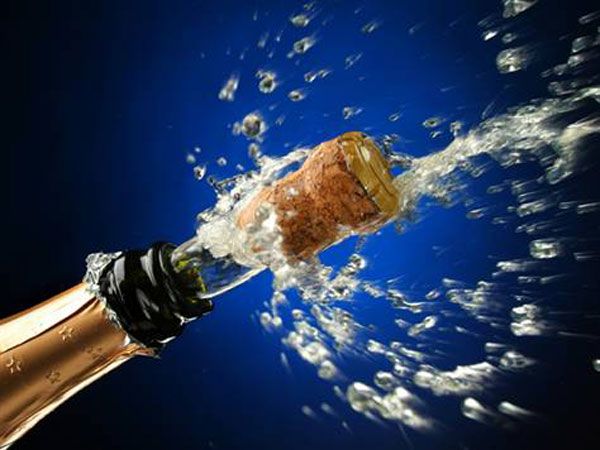A beigeish tan champagne bottle, featuring a dark green tint, is depicted popping its cork in a vibrant, dynamic close-up. Positioned from the bottom left corner, the bottle neck extends diagonally upward to the right. The gold aluminum foil around the neck, adorned with little stars, is frayed, revealing the silver underside. The cork, brown with a yellow top, is captured mid-flight about an inch from the bottle, amidst a burst of spraying champagne droplets. The background features a striking radial gradient, transitioning from a deep blue at the center to black at the edges. The overall scene is highly animated, emphasizing the explosive energy of the champagne release.